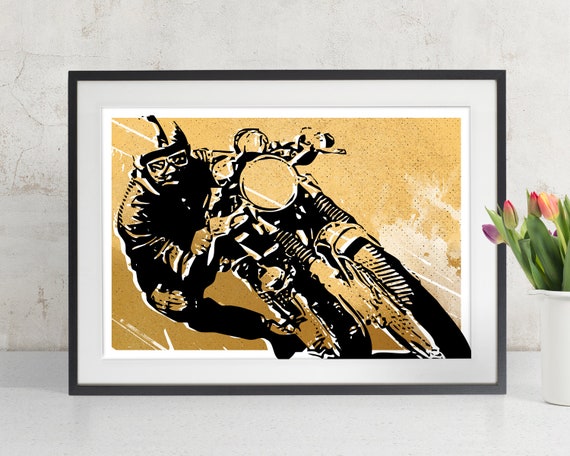The image showcases a striking piece of artwork contained within a sleek black frame. This piece, which could be either a photograph or a computer-generated image, depicts a man riding a motorcycle, captured in a dynamic pose as he leans sharply into a turn. The motorcyclist is rendered in intense black, set against a contrasting background of tannish gold, accentuated by white stripes. The artwork is neatly bordered with white edges, both directly surrounding the image and again within the frame. This visual centerpiece rests on a pristine white countertop, accompanied by a chic white vase filled with a vibrant bouquet of purple and red tulips, interspersed with fresh green leaves. The entire scene is set against a textured white concrete background, adding to the modern aesthetic of the composition.